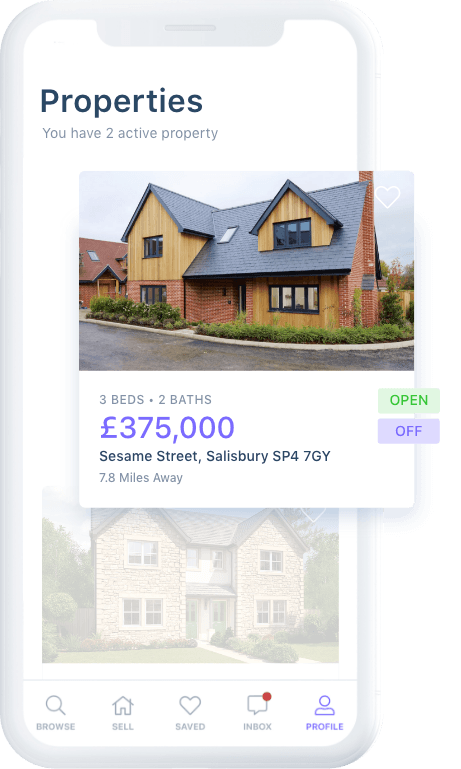The image appears to be a digital mock-up of a cell phone displayed on a white background. The phone itself, while drawn with realistic detail, does not give the impression of being a physical device that can be picked up. The smartphone's screen, also white but in a different shade, prominently features the heading "Properties" in either black or dark blue font. 

The display indicates that there are "two active properties." The first visible property listing shows a house with two peaked roofs and windows on the front. The text for this property reads: "3 beds, 2 baths, £375,000," with the address "Sesame Street, Salisbury, SP4 7GY," and its distance, "7.8 miles away." An "Open" button appears as a small green rectangle, while an "Off" button is depicted in purple. This listing occupies the primary focus of the screen, causing the second house below it to appear frosted out, signifying it is not currently active.

Beneath these property listings is the phone's navigation bar, which includes options labeled "Browse," "Sell," "Save," "Inbox," and "Profile." The overall color scheme of the image predominantly features white, black, gray, purple, green, brown, and red. There is no clear indication of the specific website or application this interface belongs to.